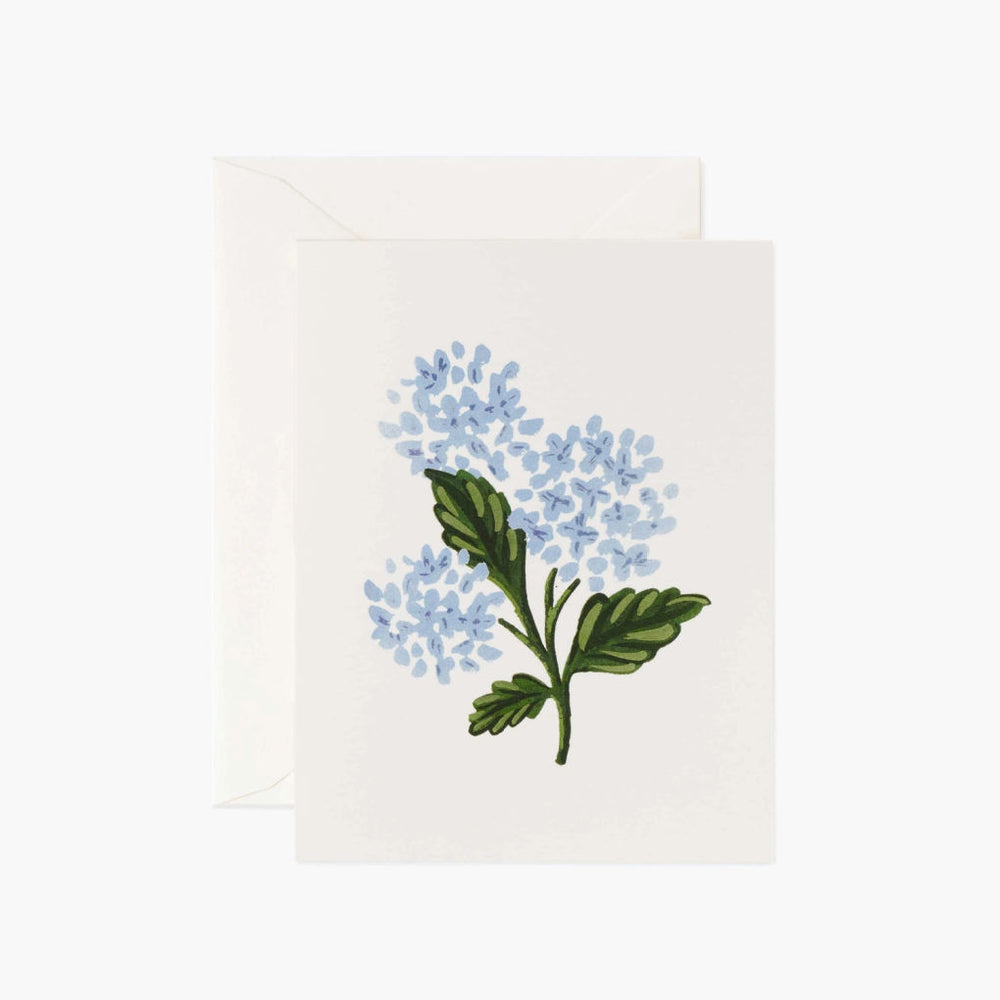The image features two posters, one overlapping the other. The visible poster on top showcases a detailed painting of blue flowers accompanied by green leaves and stems, illustrating a vibrant botanical scene. The poster beneath it is partially obscured, making it difficult to determine whether it contains any artwork. Both posters appear to be positioned against a flat surface, possibly laying on the ground or hung on a wall, though the exact setting is unclear. The visible botanical elements, including the blue blossoms and verdant foliage, are the primary focus of the upper poster, capturing a sense of natural beauty.